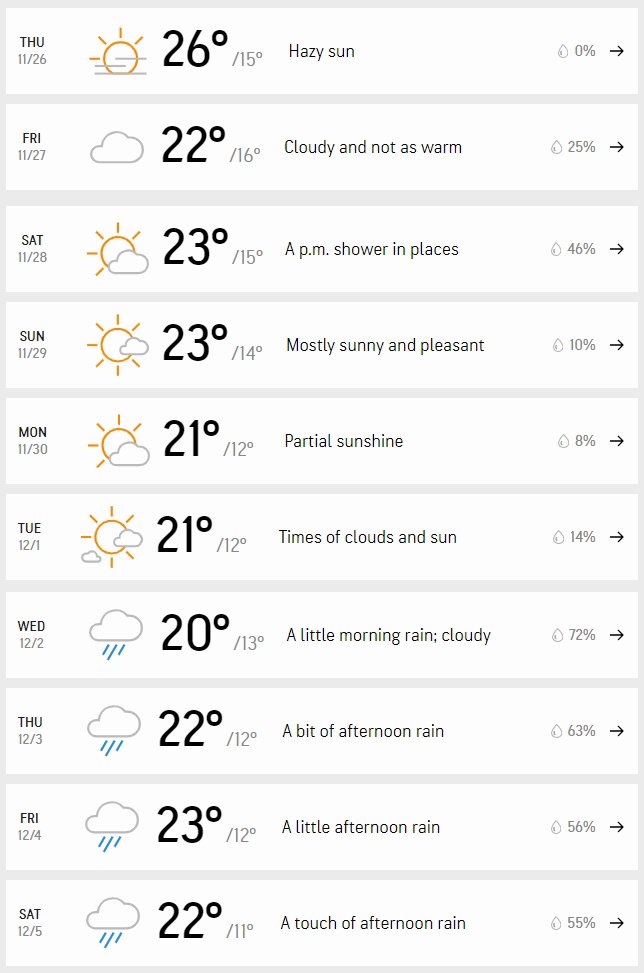This vertical, gray-bordered image resembles a weather forecast layout typical of AccuWeather.com. The forecast consists of several long, white rectangular boxes, each delineated by thin gray lines, depicting daily weather information. The high and low temperatures are prominently displayed in large black numerals, followed by smaller gray numbers. The temperature readings suggest Celsius, given that the lows are in the teens and the highs in the twenties. 

Each day is identified on the far left by a three-letter abbreviation and the numerical date (e.g., WED 12/2). The weather conditions for each day are indicated by icons—such as clouds with rain lines for rainy conditions—next to descriptive text that offers a brief summary (e.g., "a little morning rain, cold and cloudy"). To the far right, a gray raindrop icon and a percentage denote the chance of precipitation, accompanied by a small black rightward arrow. 

Between November 26th and December 5th, the forecast includes various weather conditions such as sunny, hazy, partly cloudy, and rainy, reinforcing the suggestion that this is a Celsius-based weather report from AccuWeather.com.